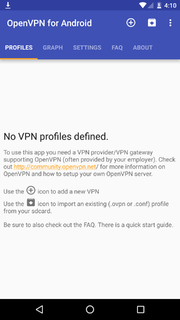**Screenshot of OpenVPN for Android Interface:**

The screenshot showcases the OpenVPN for Android app interface on a mobile device. The top portion of the app is distinguished by a blue border, prominently displaying the title "OpenVPN for Android." To the right of the title, there are two interactive icons: a circle containing a plus symbol and an ellipsis, hinting at additional options.

Below the title bar, a menu tab labeled "Profiles" spans across with a yellow underline marking its selection. Adjacent to it are additional menu options: "Graph," "Settings," "FAQ," and "About."

The primary section of the interface features a light gray background, where the text "No VPN profile defined" is displayed. This is followed by a space, leading to a more detailed instructional message stating, "To use this app, you need a VPN provider/VPN gateway supporting OpenVPN, often provided by your employer. Check out community.openvpn.net for more information on OpenVPN and how to set up your own OpenVPN server."

Another line down, further instructions are provided: "Use the circle with the plus icon to add a new VPN. Use the black square icon to import an existing profile from your SD card. Be sure to also check the FAQ; there's a quick start guide for your reference."

This detailed guide offers comprehensive steps to set up and use the OpenVPN app, ensuring users can effectively navigate and utilize its features.